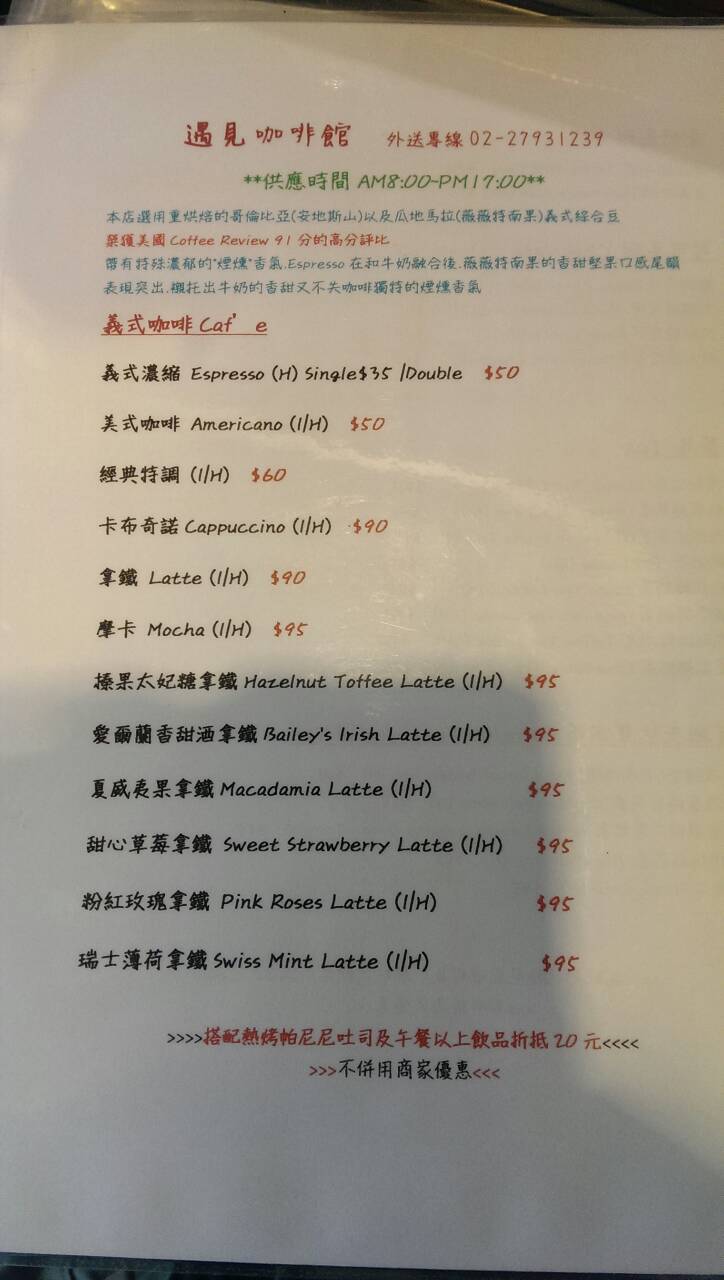The image depicts a coffee bar menu featuring both Chinese characters and English text. The menu, primarily white, prominently displays the prices in red, while the names of the items are in black. At the top of the menu, there is blue and red Chinese writing, which lacks an English translation. Below this heading, each line lists various coffee beverages — starting with Chinese characters followed by their English counterparts. The menu includes espresso, americano, cappuccino, latte, mocha, hazelnut toffee latte, and even a Baileys Irish Latte among other offerings. Notably, these items are priced quite high, with an espresso listed at $50 and a latte at $90. The hazelnut toffee latte is priced at $95, indicating a luxurious and exceptionally pricey café.